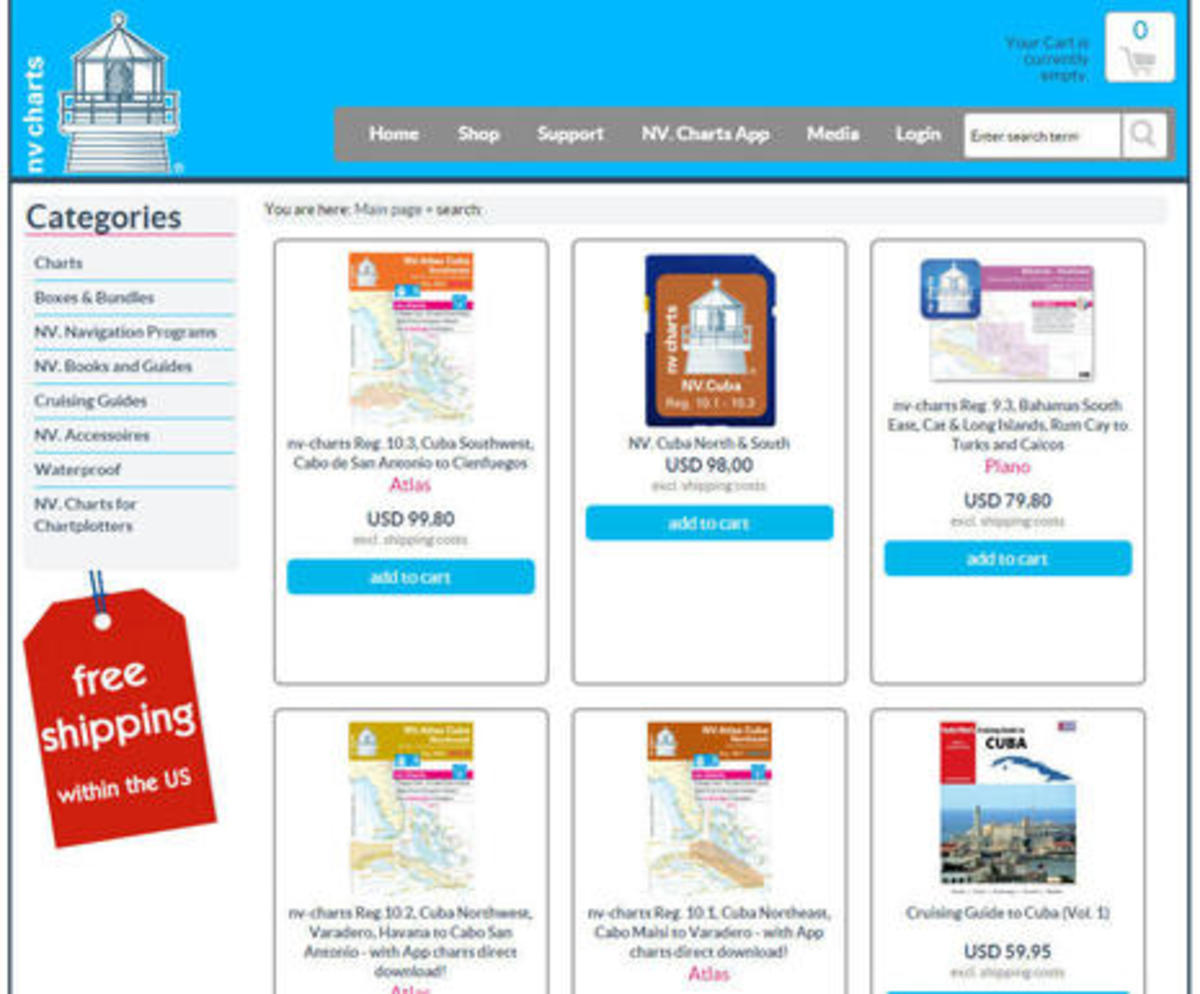The image features a webpage design with a multi-layered layout and detailed navigation elements.

At the top, the background is blue, and on the left side, the words "NV Charts" are displayed vertically, with "NV" positioned at the bottom and "Charts" above it. Adjacent to this is an illustration of a tower in white, outlined in gray.

Horizontally across the middle of the page is a light gray banner that serves as the main navigation bar. It contains the following menu items from left to right: "Home," "Shop," "Support," "NV Charts App," "Media," and "Login." Within this banner, there's a white search bar labeled "Enter Search here."

On the far right side of the gray banner, there's a cart icon indicating it is currently empty, accompanied by the text "Your cart is currently empty" with a blue '0'.

Beneath this banner, the layout is divided into various sections. On the left, the title "Categories" is boldly displayed in black, underlined by a red line. Listed below are several categories, each underlined in blue:
- Charts
- Boxes and Bundles
- NV Navigation Programs
- NV Books and Guides
- Cruising Guides
- NV Accessories
- Waterproof
- NV Charts for Chart Plotters

To the right, there is a prominent red tag reading "Free Shipping within the US."

The main content area is divided into two sections of product listings. The top row comprises three products outlined in gray:
1. The first product titled "Atlas," priced at USD 99.80, includes a blue "Add to Cart" button and an image of an Atlas book.
2. The second product is "NV Cuba North and South," priced at USD 98, also with an "Add to Cart" button.
3. The third product is labeled "Piano" in pink, priced at USD 79.80, with an "Add to Cart" button. Above these products, there's a blurry description mentioning "Bahamas South" and "Long Islands, Ryan City to Turks and Caicos."

The bottom row features another set of three products, but they are partially cut off:
1. The leftmost product appears to be an Atlas, though its details are blurry.
2. The middle product similarly has "Atlas" in its description but is blurry.
3. The final product clearly states "Cruising Guide to Cuba, Volume 1," priced at USD 59.95, with a blue line that is also cut off at the bottom.